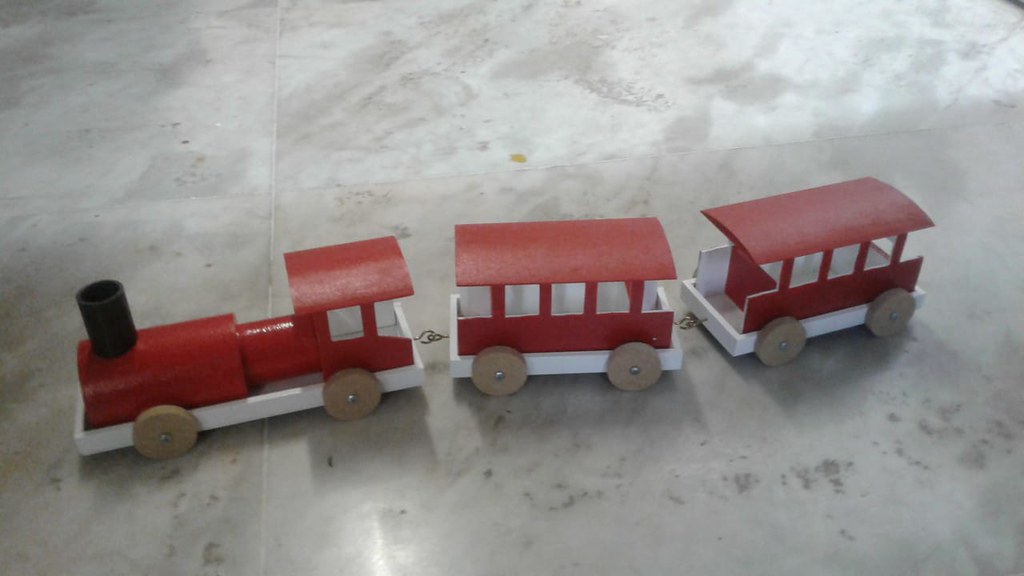The image features an antique, handcrafted wooden toy train placed on a white marble-tiled floor. The vintage train set is painted a striking red with a white bottom and interior, and it includes three segments—an engine and two carriages—connected by silver clasps and hooks. Each component has wheels left in their natural light brown wood color. The engine sports a distinctive black smokestack, while each carriage has five windows. Although unoccupied, the carriages are designed to potentially hold small toys or dolls, making it an ideal plaything for a child. The train's meticulous craftsmanship and classic design suggest it's a cherished toy meant to be handled with care.